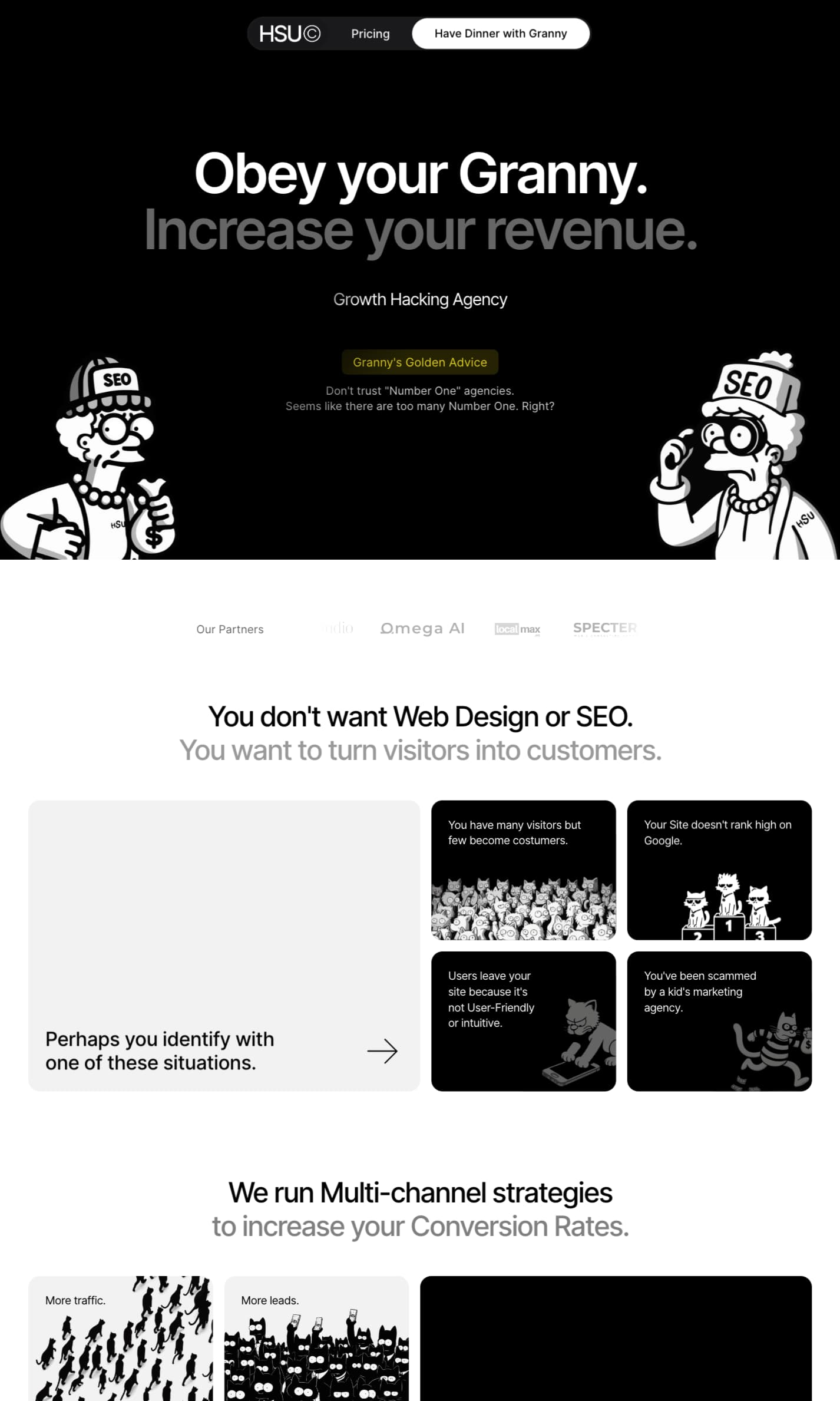**Website Description: "Obey Your Granny" Digital Marketing Agency**

The website features a striking black-and-white design with minimal use of color for emphasis. The layout is in portrait mode, making it well-suited for mobile viewing. At the top, a solid black background houses the main navigation elements. In bold white letters, "HSU" is prominently displayed, and adjacent to it, the word "Pricing" is partially visible. Also, there is an oval-shaped search bar integrated within this section, offering functionality to the user.

Taking center stage is the bold slogan, "Obey Your Granny," printed in large, white font. Just below, in smaller gray text, the phrase "Increase Your Revenue" is designed to catch the eye. 

Further down, the phrase "Something-or-other Hawking Agency" is visible, followed by two distinct illustrations of elderly women, each drawn in the recognizable style of Matt Groening, the creator of The Simpsons. The old lady on the left dons a white, boxy hair accessory labeled "SEO" and holds a money bag, along with a string of pearls around her neck. On the right, another elderly woman, also wearing pearls, is depicted with a pair of goggles.

Continuing down the page, a section with a white background addresses the viewer directly with the statement: "You don't want web design or SEO. You want to turn visitors into customers." Following this declaration, the website invites visitors to identify with one of several situations listed below.

Four thumbnail-sized illustrations follow, each radiating the iconic Simpson-esque style. These appear white against the black background. Each illustration depicts three distinct scenarios primarily involving cat figures: one featuring three cats, another showing a crowd of cats, a cat burglar clad in stripes, and finally, another crowd scene which likely consists of cats as well. Each illustration has accompanying blurbs offering further context.

The concluding section of the page states, "We run multi-channel strategies to increase your conversion rates," rounding off the page with a promise of comprehensive marketing strategies aimed at enhancing customer engagement and conversion.